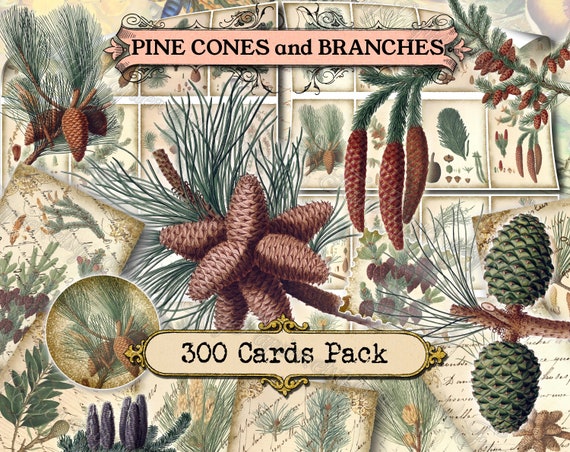This is a highly detailed advertisement for a pack of playing cards showcased on the packaging. The front of the pack prominently displays text indicating "300 cards per pack," immediately informing potential buyers of the substantial quantity included. The text "icons and branches" is also visible, hinting at the artistic theme featured on the cards themselves. True to this description, the entire cover is adorned with intricate illustrations of various icons and branches, offering a visual preview of the creative design that awaits inside.

Adding a unique touch, the bottom left corner of the packaging features a perfectly cut circular window. This design element allows consumers a sneak peek into the card center within the packaging, exemplifying the quality and style of the cards enclosed. Combined, these detailed visual and textual elements make a compelling first impression, enticing customers with both quantity and artistic flair.